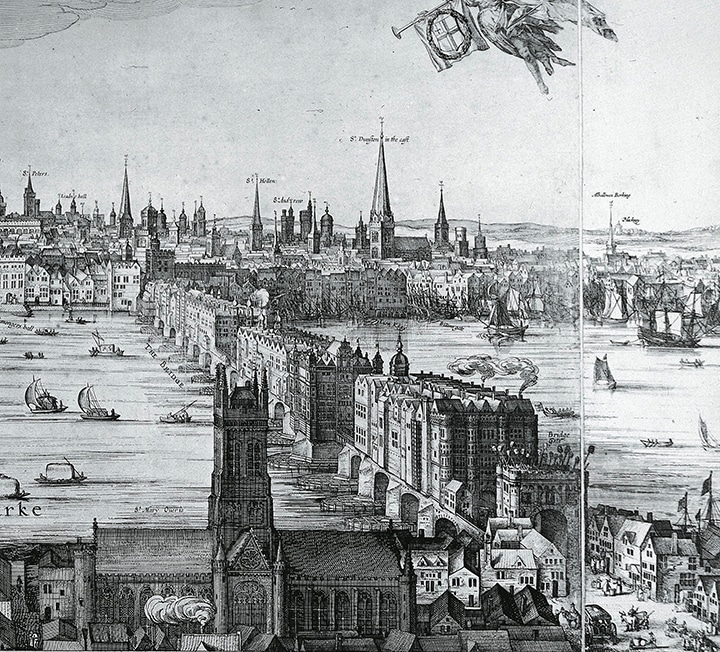This black and white illustration appears to depict a historic European city situated along a waterfront. The drawing is highly detailed, showcasing an array of tall, medieval-style buildings with pointed steeples, some of which have indecipherable labels above them. On both the left and right sides of the image, bodies of water are visible, populated with numerous boats navigating through channels that run beneath bridges connecting various parts of the city. Towards the top section of the image, a cherub-like figure or bird-like creature holding an object hovers in the sky, adding a whimsical touch. In the background, smoke can be seen rising from what seems to be one of the ships, hinting at a bustling, industrial vibe. The overall quality of the illustration suggests it may have been intended for a book or similar publication.